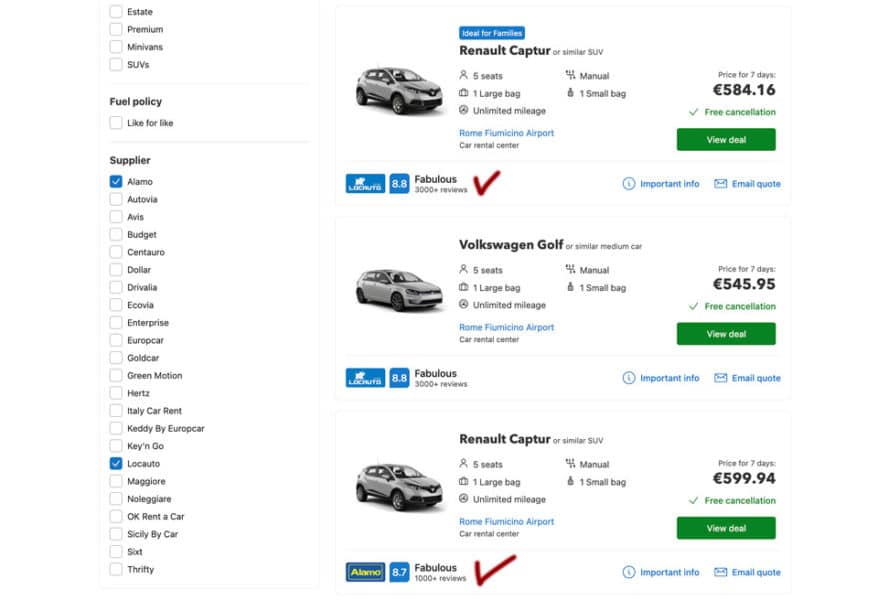The screenshot features a comparison of three light gray SUVs against a white background. The first vehicle, identified as a Renault Captur, is listed with a price of $584.60 pesos. The second vehicle, a Volkswagen Golf, is marked with a red check and priced at $545.00 pesos. The third vehicle, another Renault Captur, is listed with a price of $599.00 pesos. Each option includes a "View Deal" button, which is a green rectangle featuring the text "View Deal" in green. To the left of each listing, there is information regarding the fuel policy and the supplier, presented with checkboxes. Notably, the checkbox for Alamo is checked, alongside other suppliers such as Lakuto LLC AUTO.